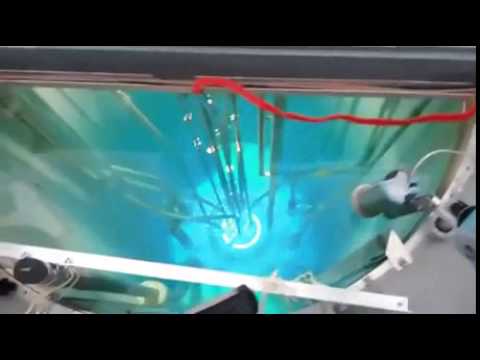The image captures a see-through water tank from an above-facing vantage point. The tank contains light blue water with a greenish hue, appearing bluer in the center and greener towards the edges. Large reeds or poles extend from the bottom to the top of the water, while bubbles can be seen rising from the cables below, suggesting an aquatic environment. A prominent red wire runs across the top of the image, connected to the tank, though its function is unclear. On the right side of the tank, an electronic device, likely a camera, appears to be filming the interior. A thin white beam extends from the left side to the bottom right corner, and a white metal bracket is visible at the bottom of the pane. Outside the tank, fixtures include a white wall to the right and a dark gray or blue header above it.